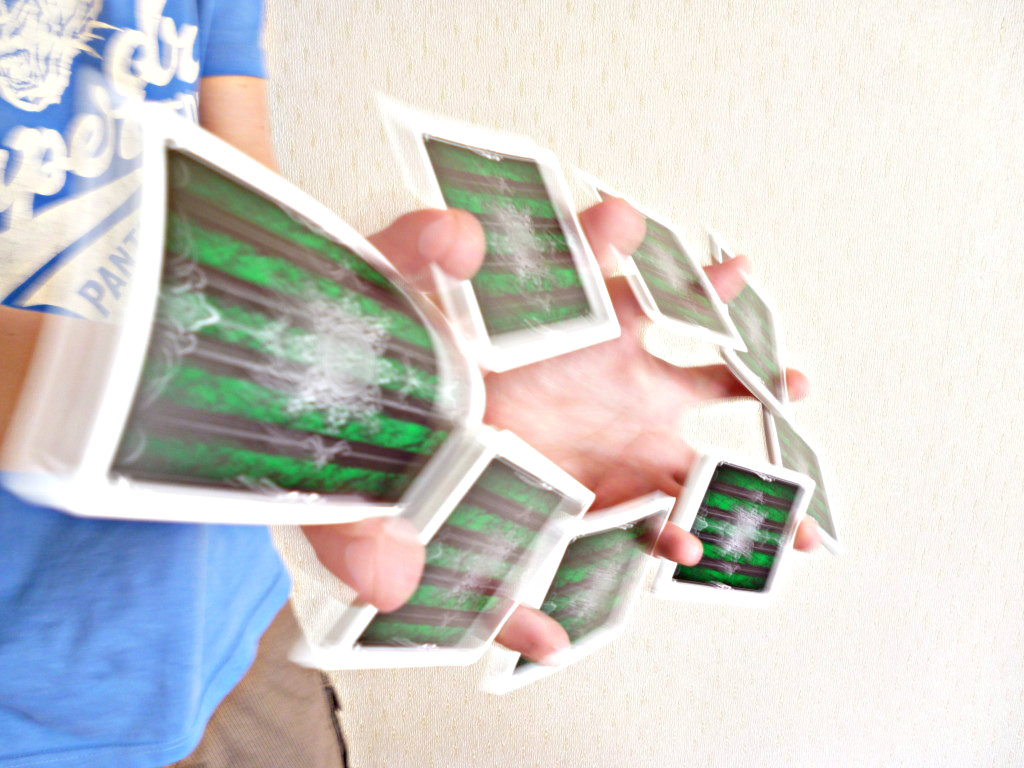A captivating image captures the dynamic motion of an individual performing a card trick. Positioned on the left edge of the frame, the person, dressed in a blue shirt adorned with a white graphic design resembling the name of a team or city with an underline, commands attention. Although only a hint of their brown pants is visible, the shot primarily focuses on their chest and neck area, emphasizing their actions. The magician's hands, emerging from the left side of the photograph and extending diagonally to the right, are deftly positioned wrist to wrist. Cascading between their fingers are small piles of playing cards, all face down in a fascinating display of dexterity. The cards, characterized by white borders encircling green rectangles adorned with black vertical lines interspersed with thin gray lines, add to the visual intrigue. This remarkable feat is set against a clean, white background wall, further highlighting the complexity and skill of the card trick in a perfectly timed freeze-frame.